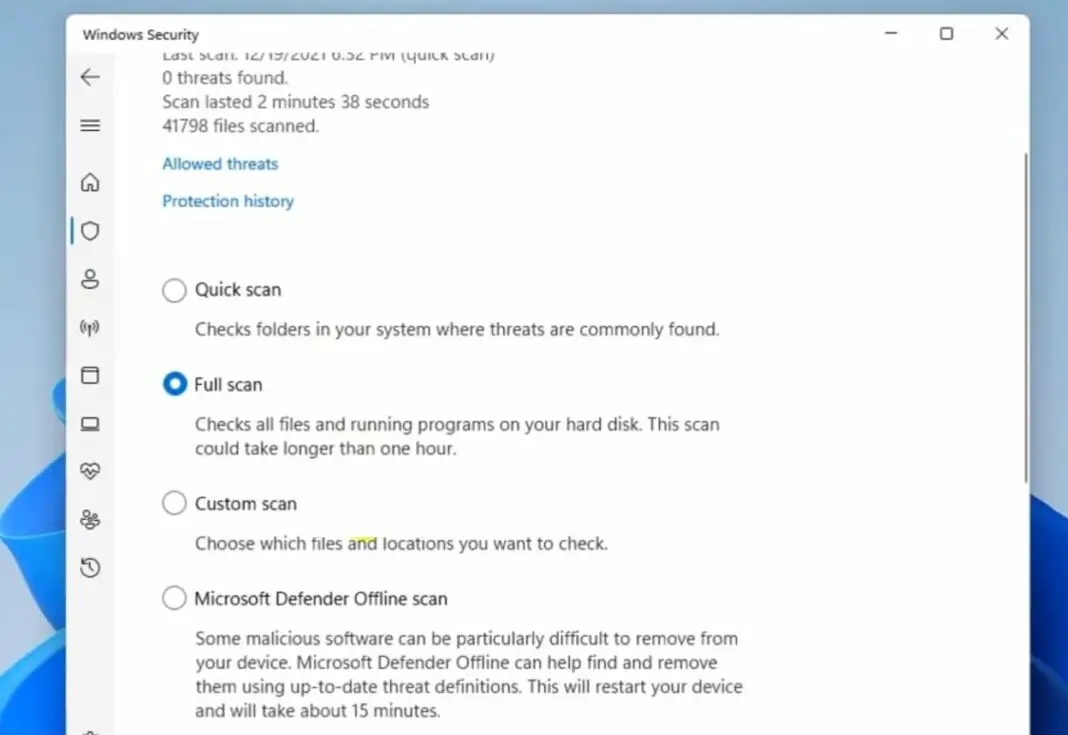This detailed screenshot captures a desktop display on a Windows computer, prominently featuring the Windows Security program interface. The top of the window hosts standard control buttons: minimize, maximize, and close (X). On the left side, a vertical menu features a series of icons: an arrow pointing left, the hamburger menu (three lines), a house icon, a shield, a generic head-and-shoulders figure, an antiquated wireless access point symbol, a box, a laptop, a heart resembling a hot air balloon, a flower, and a clock indicating backward time.

At the top of the main window, it states, "Last scan: December 19, 2021, at [time] 52 PM," with a summary beneath: "Quick scan: zero threats found. Scan lasted 2 minutes and 38 seconds. 41,798 files scanned." Two clickable blue links are visible: "Allowed threats" and "Protection history."

Various scan options are detailed for selection: 
- **Quick Scan:** Checks folders in your system where threats are commonly found.
- **Full Scan** (currently selected): Scans all files and running programs on your hard disk; this can take longer than an hour.
- **Custom Scan:** Select specific files and locations to check.
- **Microsoft Defender Offline Scan:** Designed for removing particularly stubborn malware, this option uses the latest threat definitions and requires a device restart, taking approximately 15 minutes.

This screenshot clearly illustrates the Windows Security settings and options available for thorough system protection.